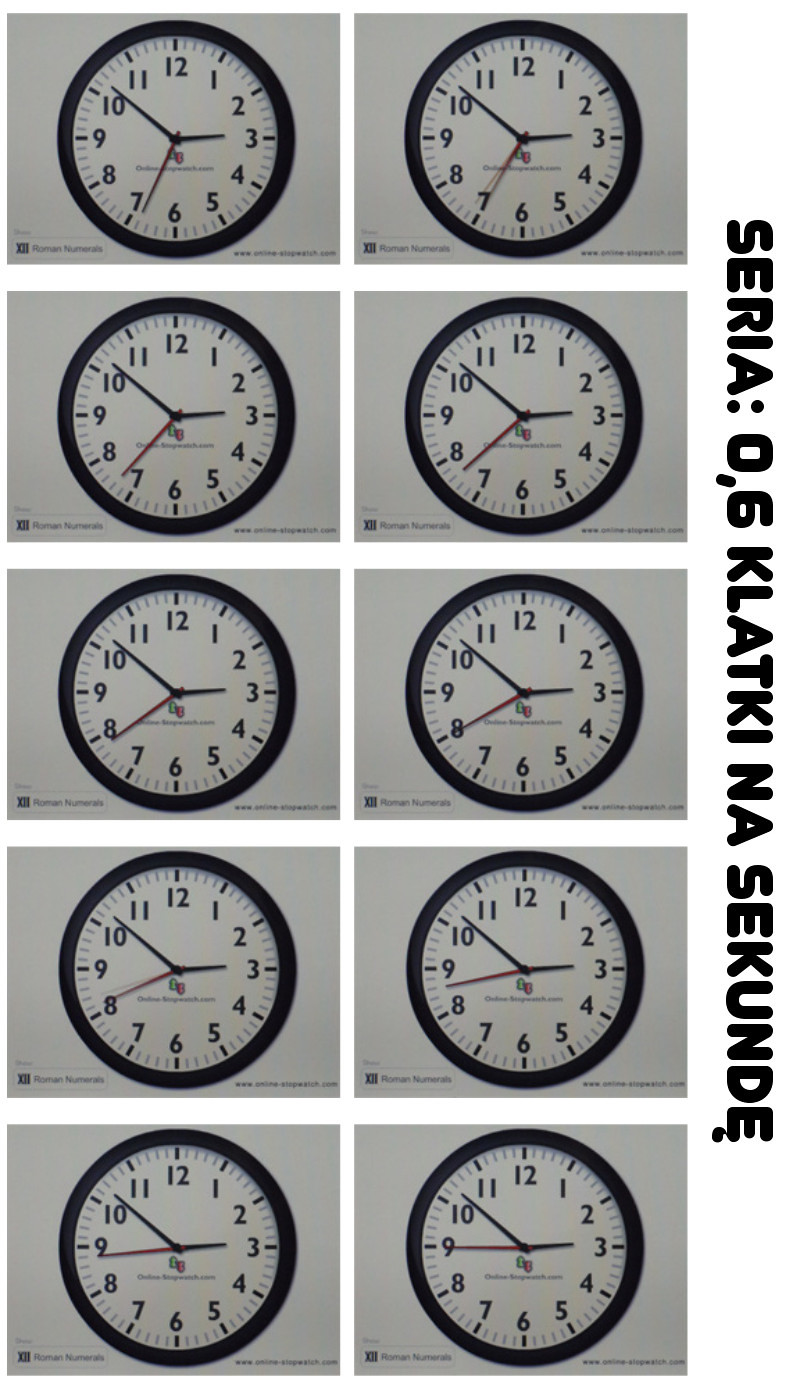The image is a meticulous grid layout consisting of ten individual clock faces, arranged in two vertical columns and five horizontal rows. Each clock face vividly displays black numerals and black hour and minute hands, set against a clean white background with a black border. Notably, the red second hand varies across each clock, showing incremental movements to capture different moments in time. The clocks consistently display the time as approximately 8 minutes to 3 o'clock. Beneath each clock lies an indistinguishable black print on a greyish rectangular background. Along the right-hand side of the grid, a non-English vertical inscription reads "SERIA: 0.6 KŁATKI NA SEKUNDĘ." This meticulous arrangement and subtle movement capture a dynamic and precise visual representation of time.